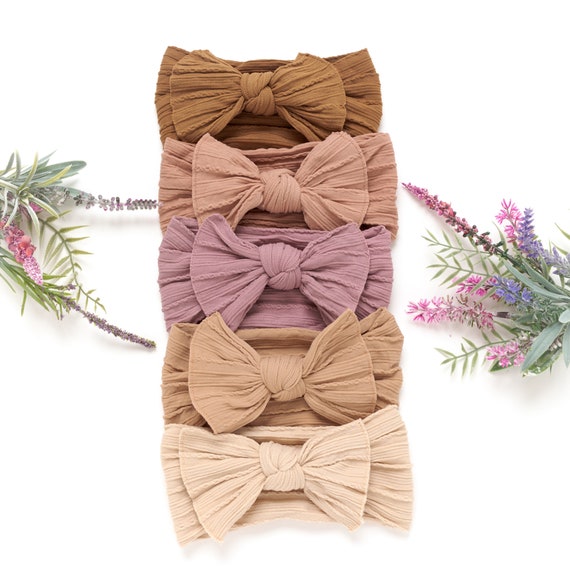The image features a vertical stack of five bow ties centrally placed against a white background. The bow ties are arranged in a descending order of colors: brown, pale pink, light purple, beige, and white. Each bow tie is tied neatly in the middle, showcasing a soft, crepe-like fabric. Flanking either side of the bow ties are delicate bouquets containing flowers in shades of pink to lavender, complemented by pale green leaves. These floral accents add a decorative touch, highlighting the pastel and neutral tones of the bow ties, alluding to an overall theme of fashion accessories, potentially targeting a female audience.